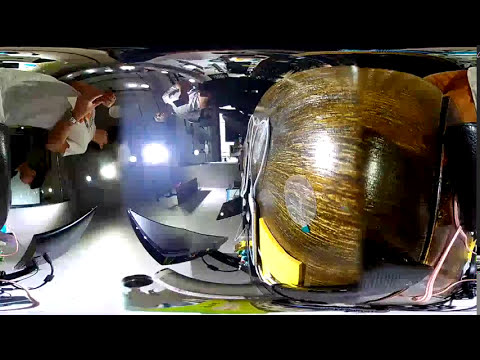This perplexing image presents a 360-degree fisheye panoramic view, possibly digitally stitched together, resulting in a highly distorted perspective. The composition includes a mixture of objects and people within what appears to be an interior room. On the right side dominates a large, spherical, glossy wooden object with dynamic shades of browns and yellows that could either be a wall or some unique furniture piece due to the odd distortion caused by the lens. 

Towards the upper left corner, a man in a short-sleeve white T-shirt, with bare arms and potentially a pencil in his left hand, appears to be floating, although this could just be an artifact of the camera angle. His actions are blurred, making his head unclear. Additionally, there are various light sources and panels throughout the image, including what seem to be LED or LCD screens.

Elsewhere, a computer monitor is distinctly visible in the lower left corner, and possibly other laptops are scattered around, adding to the room's high-tech vibe. The lower right corner features something pink, perhaps a cord. The overall warped and confusing nature of the image makes it challenging to decipher the exact setting, but it certainly blends elements of a home or office with futuristic, almost spaceship-like qualities.